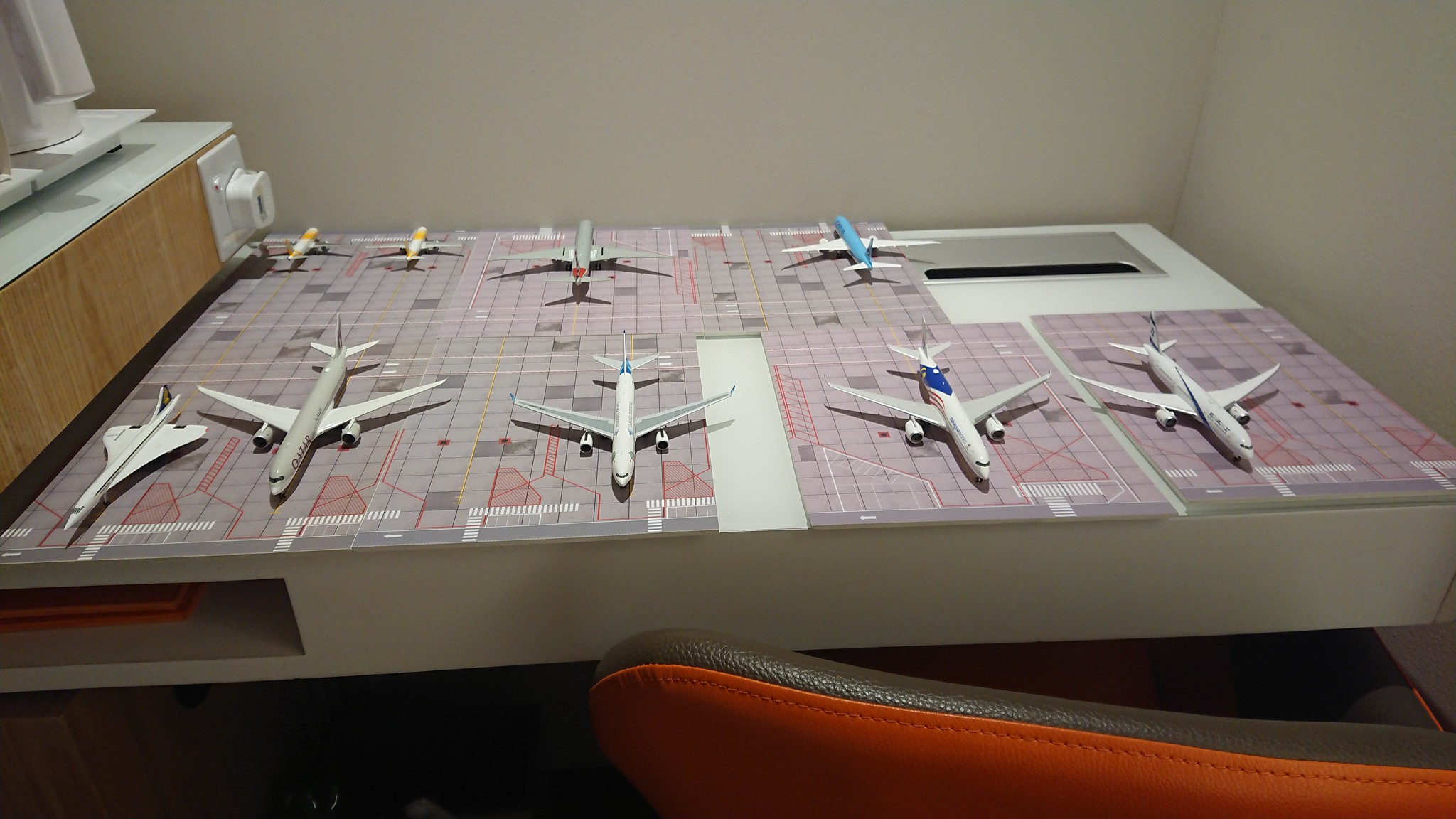This image showcases a detailed model airport scene set atop a grid-lined platform with light pink and darker colored lines, giving the impression of a runway. The scene features nine miniature commercial jets of various sizes and designs, meticulously arranged in two rows: five planes facing the viewer in the front row and four planes oriented away in the back row. 

Among the colorful array of model planes, notable designs include a red, white, and blue plane, a plane with blue and white wings, a gray plane with white wings, and two smaller planes with yellow, white, and black markings. Additionally, there is a white plane with blue patterns, a tan plane with orange accents, and a light gray plane with white wings.

The setting appears to be a tabletop in a room with white or beige walls, adding to the complexity of the scene. A notable piece of furniture is the orange and brown chair visible in the foreground, providing a sense of scale and context to this detailed miniature airport display.